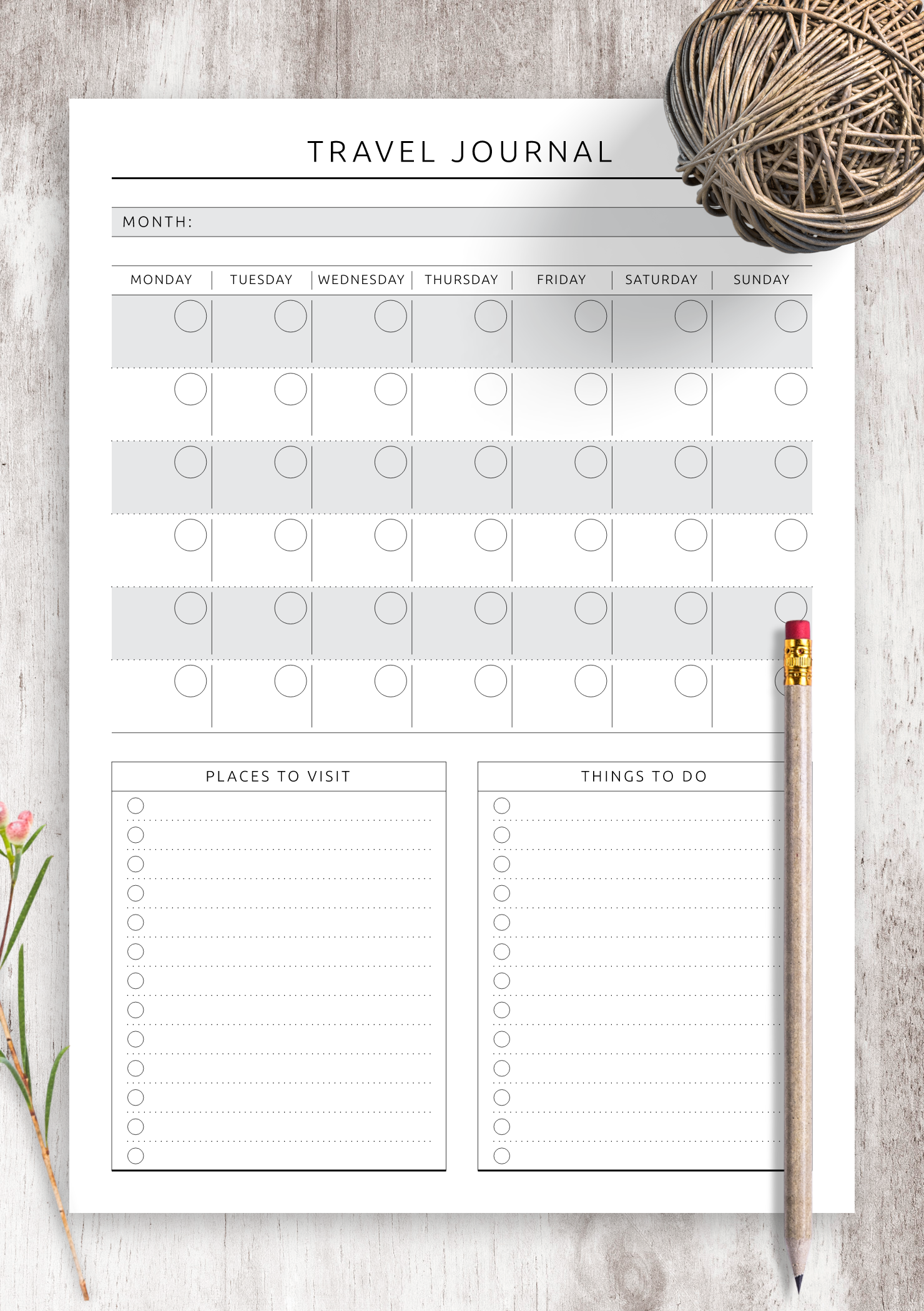This image captures a well-organized page from a travel journal, placed on a grey wooden table. The top of the journal page features a light grey box labeled "Month," where travelers can jot down their travel month. Below this, there is a well-structured calendar spread across six rows and seven columns, each column representing a day of the week from Monday to Sunday. Each day in the calendar alternates in grey and white strips, with small circles in the top right corner of each day for check marks or notes. 

Beneath the calendar, on the left side of the page, is a section titled "Places to Visit," which includes lines for entering destinations and small circles next to each line for ticking off visited places. On the right side, there's a similar section titled "Things to Do," designed in the same format with lines and tick circles. 

The journal page is held down at the top right by a ball of twine, adding a rustic charm. At the bottom right of the page lies a wooden pencil with a shiny gold tip and a pink eraser, ready for use.